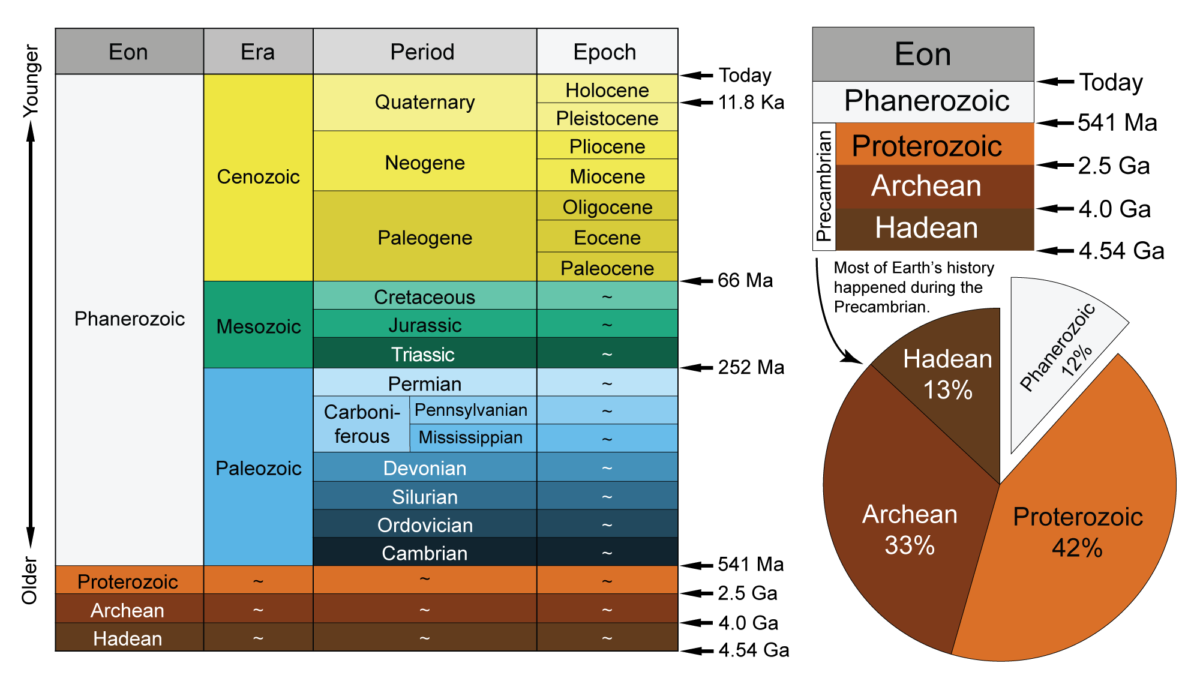This image is a detailed chart that depicts the geologic time scale of Earth's history on a white background. On the left side, there is a large vertical timeline with an arrow pointing up labeled "younger" and pointing down labeled "older." At the top of this timeline, it categorizes time into Eon, Era, Period, and Epoch. The primary Eons listed are Phanerozoic, Proterozoic, Archean, and Hadean. Each Eon is further divided into Eras, such as the Cenozoic, Mesozoic, and Paleozoic, as well as into various Periods including the Neogene, Paleogene, Jurassic, and Devonian. This colorful timeline features various colored bars—yellow, green, blue, orange, red, and brown—to distinguish between different segments of Earth's history, with corresponding numerical data on the left side.

In the bottom right corner, there is a pie chart breaking down the percentage of Earth's history each Eon represents: Phanerozoic (12%, white), Hadean (13%, brown), Archean (33%, various colors), and Proterozoic (42%, various colors). Above this pie chart, another small square graph displays colored bars representing Eons with related numerical data. Overall, the chart provides a detailed and colorful visualization of Earth's geologic history, emphasizing the distribution and duration of different Eons and Eras through intricate diagrams and data.